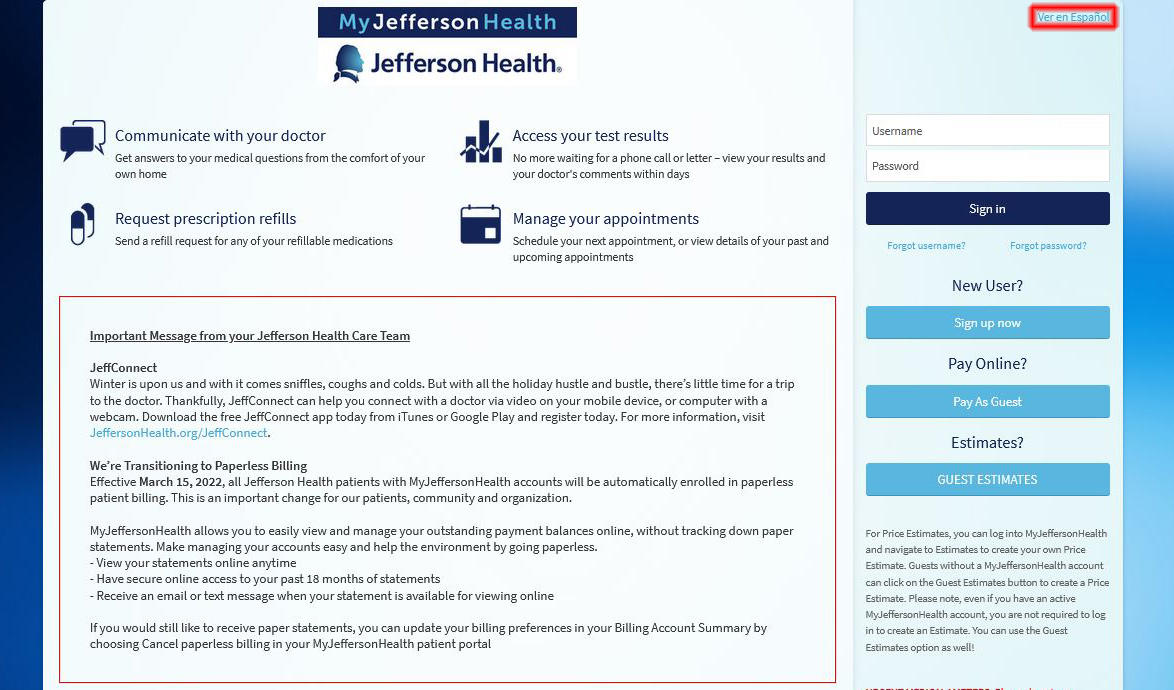Screenshot Description:

The image is a landscape-oriented screenshot from a web page, possibly displayed on a laptop or a monitor. The design features distinct blue borders on both the left and right sides, creating a visually balanced frame. The left border starts with a nearly black shade at the top, transitioning to a medium intense blue towards the bottom. In contrast, the right border is light blue at both the top and the bottom, with a medium blue section in the middle.

The central header of the webpage reads "My Jefferson Health," with "My" and "Health" in blue and "Jefferson" in white, set against a very dark blue or black bar. Adjacent to this text is the Jefferson Health logo, depicting a silhouette of Thomas Jefferson's head, accompanied by the words "Jefferson Health."

Below the header are four informative sections, each with an icon and a brief description:

1. **Communicate with Your Doctor**: Represented by overlapping speech bubble icons, this section invites users to get answers to their medical questions from the comfort of their own homes.

2. **Access Your Test Results**: Illustrated with a bar graph and an overlaid zigzag graph, this section informs users that they no longer need to wait for phone calls or letters; they can view their results and doctor's comments within days.

3. **Request Prescription Refills**: Featuring an icon of two medication capsules, this section allows users to send refill requests for any of their refillable medications.

4. **Manage Your Appointments**: Displayed with a calendar icon, this section enables users to schedule their next appointment or view details of past and upcoming appointments.

A rectangular block of text with a thin red outline provides an "Important message from your Jefferson Health Care team." The content mentions the transition to paperless billing and other updates under the "Jeff Connect" initiative.

To the right of the image, before reaching the light blue border, is a light blue column housing the login page. This section includes fields for username and password with a "Sign In" button underneath. Below are additional options with three light blue buttons: "Sign up now," "Pay as guest," and "Guest estimates," catering to new users and facilitating online payments and service estimates.